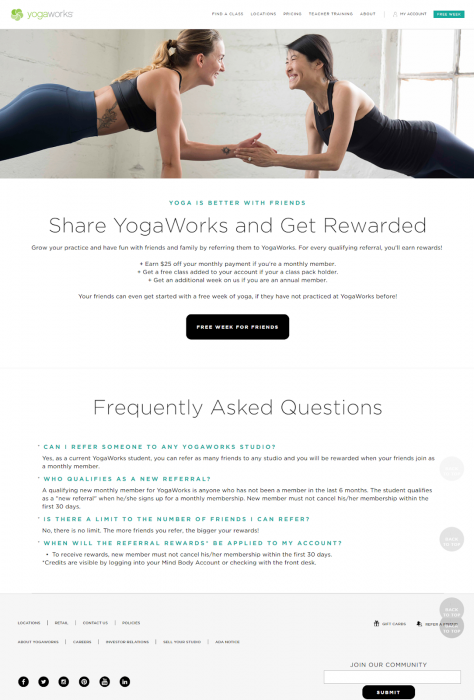Discover a world of yoga at YogaWorks! Our Macau locations offer a variety of classes and training sessions in serene environments. Imagine a vibrant studio featuring a charming brick wall and sunlit windows. In the foreground, a joyful yogi, adorned with tattoos, strikes a pose in a form-fitting tank top and pants, showcasing the harmony of strength and flexibility. The welcoming atmosphere highlights the belief that yoga is better with friends—share your YogaWorks experience and reap the benefits!

Become a part of our community and enjoy exclusive rewards. Monthly members can save $25 on their payment by referring friends. Class pack holders receive an additional week, and new members starting with a free week can spread the joy by earning a free week for a friend.

Our FAQ section explains that current students can refer friends to any YogaWorks studio with no limit on the number of referrals. More referrals mean more rewards! Note that referral benefits kick in only if the new member maintains their membership for at least 30 days. Grow your practice, bond with friends, and get rewarded with YogaWorks!